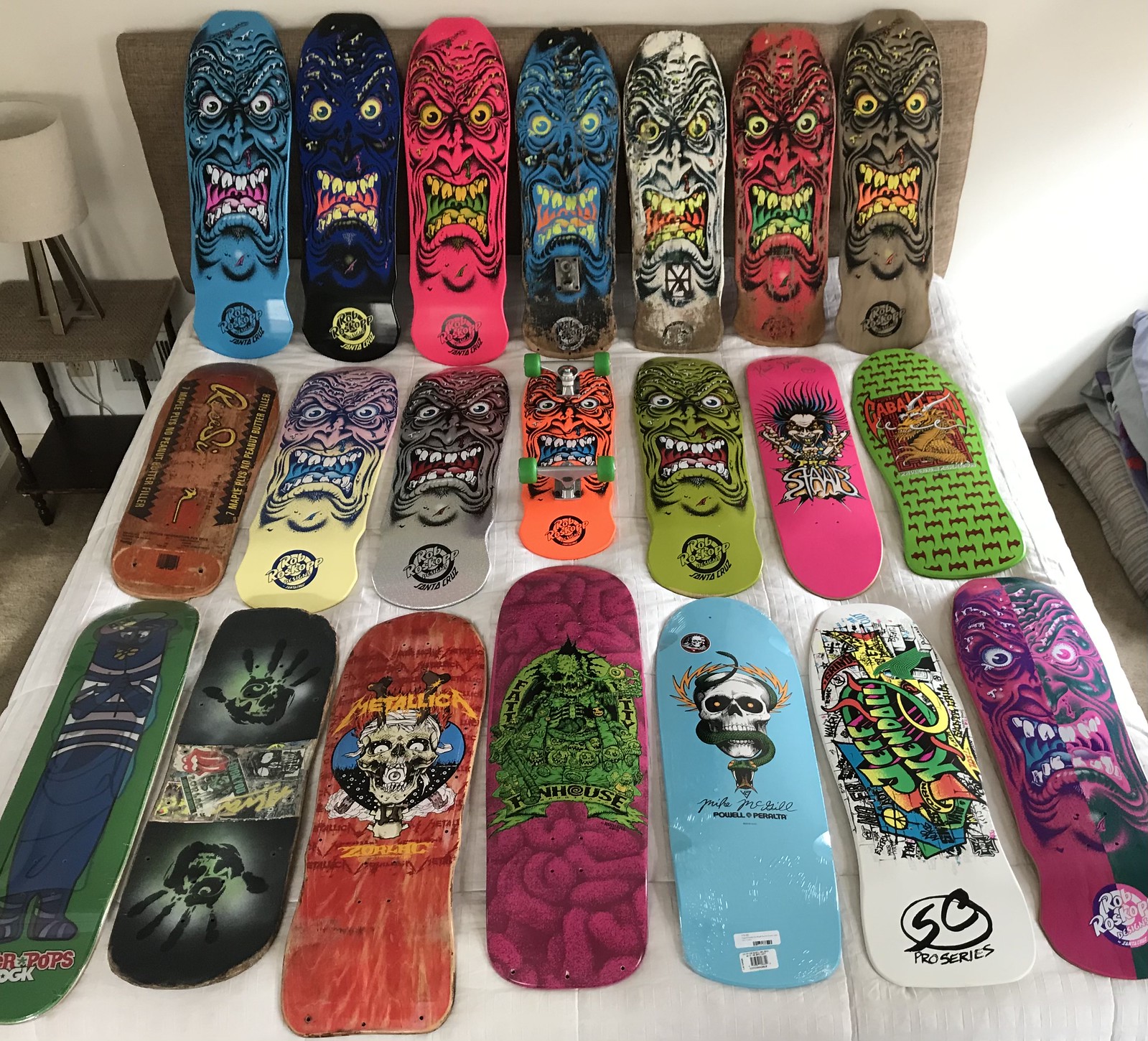In this image, there are three rows of skateboards arranged on a white cloth or blanket. The skateboards, most of which have no wheels attached, showcase their intricately painted undersides with a variety of eccentric designs. The top row is leaning against a headboard-like structure covered in brown linen, resembling a headboard in a bedroom or a cushion in a store display. This row prominently features menacing faces with yellow teeth. The middle row includes a skateboard with green wheels and silver wheel holders, while the rest lie flat, showcasing designs such as skulls, crossbones, and a "Metallica" logo. The skateboards display a colorful array of hues, including blue, purple, pink, white, brown, green, orange, and red. In the background, a white wall is flanked by side tables, one of which holds a lamp with a white lampshade, lending a cozy, yet eclectic atmosphere to the setting.